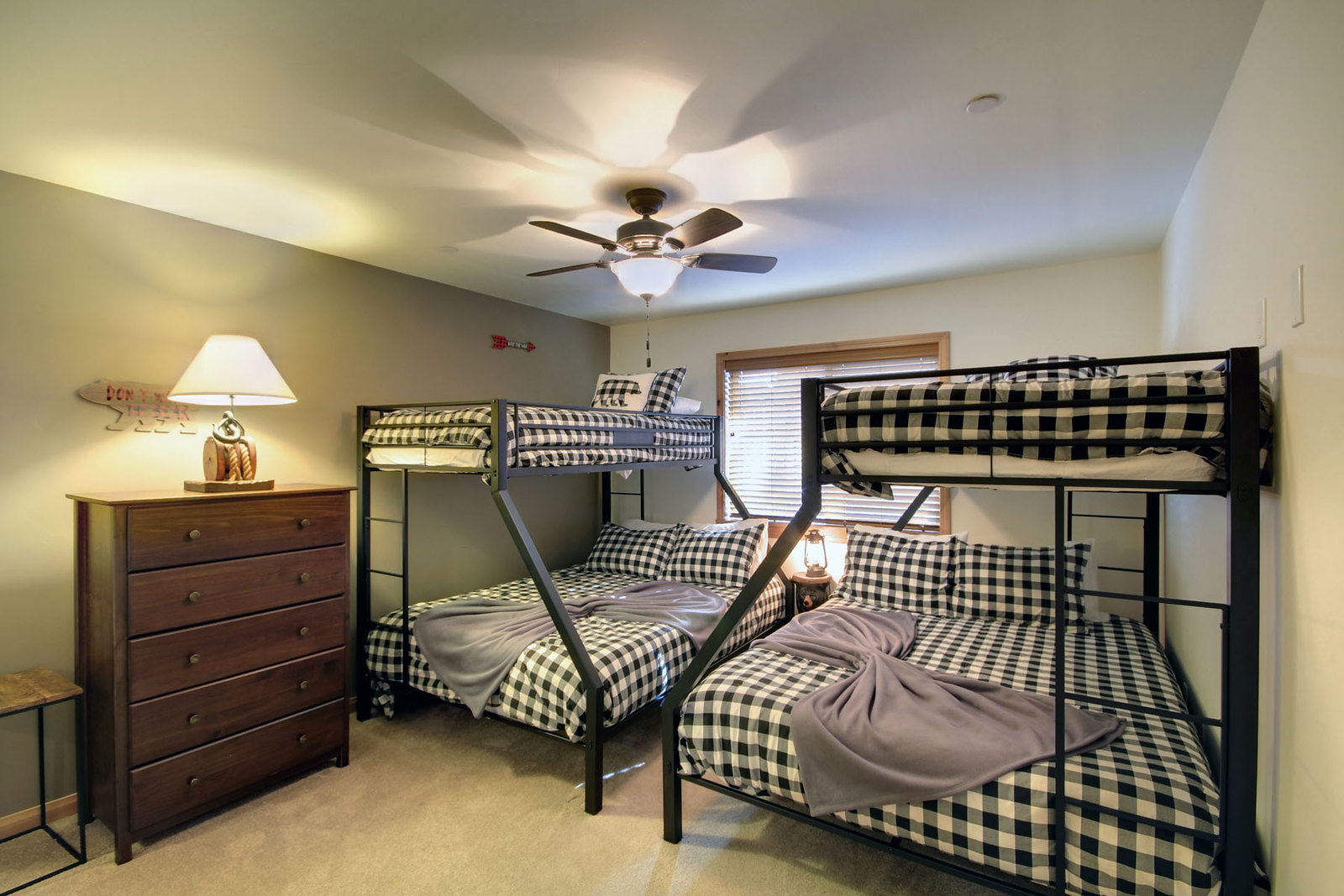This color photograph captures the interior of a bedroom, viewed through the door with a potential wide-angle lens. Central to the image are two adjacent bunk beds framed in black lacquered metal. Each bunk bed features a double bed on the bottom and a single bed on the top, with ladders positioned for access. The beds are dressed in black and white gingham print sheets, with the bottom bunks showcasing two matching pillows and light purple blankets arranged in an hourglass pattern, while the top bunks have one pillow each. 

A ceiling fan with an illuminated light is mounted in the center of the ceiling. The room's walls are a light cream color, complemented by a cream-colored carpet. To the left of the bunk beds, a dark wooden chest of drawers stands against the wall, topped by a large lamp that is also turned on. Behind the beds, a window with a wooden frame and white blinds allows natural light to filter into the room. The overall layout and decor suggest a cozy, neatly arranged bedroom, possibly intended for children or guests.